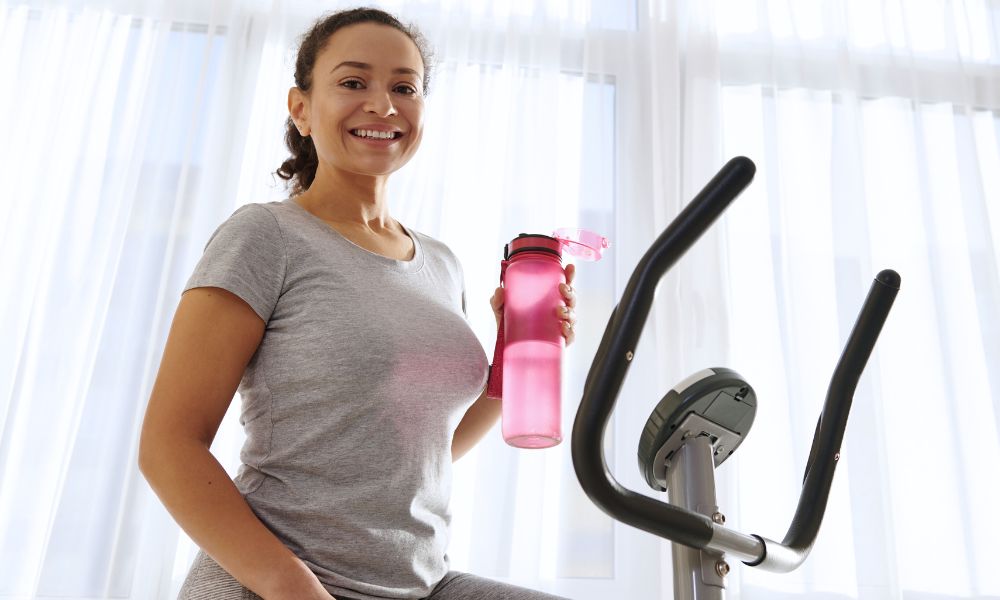The indoor photograph captures a woman smiling widely at the camera while mid-exercise on a stationary bike. Her light brown skin glows in the natural sunlight streaming in from a window behind her, covered with semi-transparent white curtains. She has shoulder-length curly brown hair that is brushed back, and she is dressed in a light gray t-shirt paired with slightly darker gray sweatpants. In her left hand, she holds a pink workout water bottle with an open lid. The exercise bike she's seated on features a silver neck with black handlebars and a circular electronic display unit, suggesting sophisticated design. The setting is bright and airy, with the woman exuding happiness, readiness, and positivity, possibly indicative of a fitness advertisement.